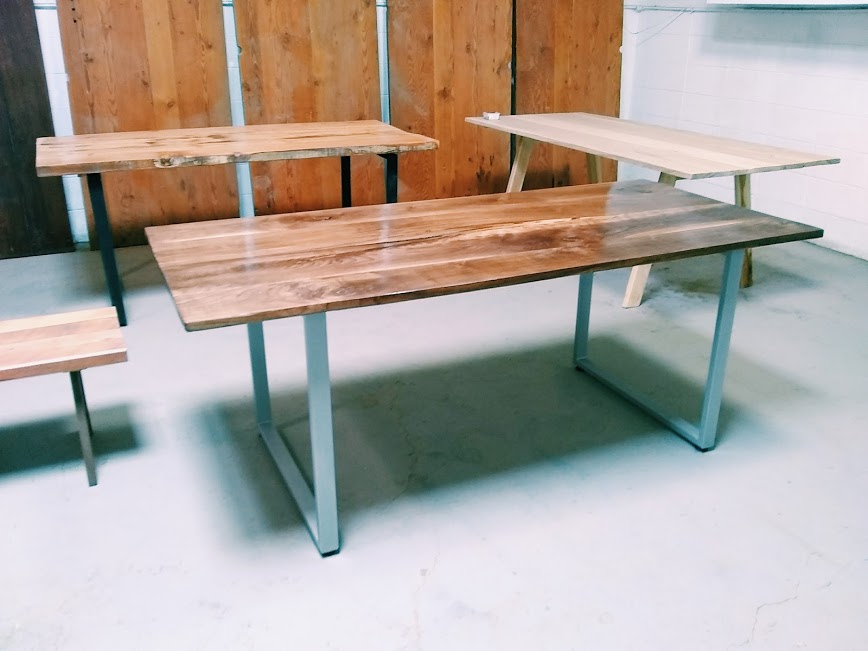The color photograph captures an indoor room featuring a series of wooden tables with varied designs and colors displayed on a floor with a marble effect. The floor predominantly features white and dark grey striations. The lighting from above casts distinct shadows of the tables beneath them. Positioned in the foreground, one table showcases a dark mahogany surface with U-shaped metal legs. In the back left, another table with a wooden surface rests on triangular black metal legs, presenting a contrasting style. The table in the back right has a pine-colored wooden surface with matching wooden legs. 

To the left side of the room, a small wooden bench is present, and four large pieces of treated and finished wood, dark brown with orange and red accents, lean against the pristine white wall. Next to this cluster of planks is a dark brown, nearly chocolate-colored wooden door. Overall, the room's composition showcases a sophisticated assortment of wooden furniture and woodworking elements, highlighted against a minimalist backdrop.